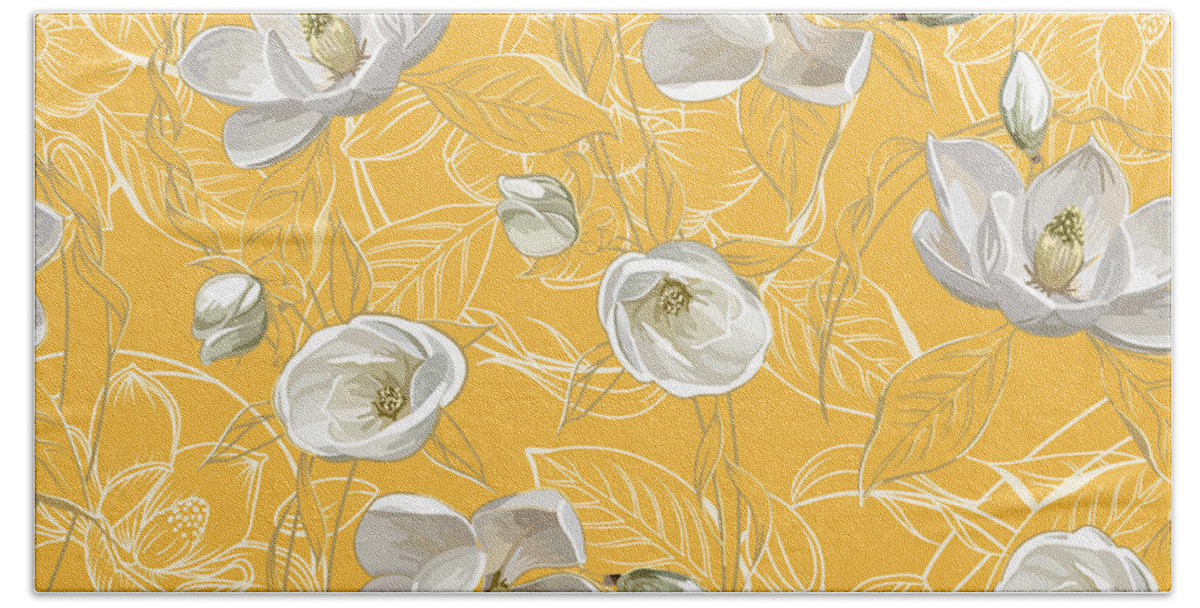The image is a close-up of a rectangular section of wallpaper with a soft orange-yellow background, featuring large white flowers that appear highly three-dimensional due to their detailed shading and white highlights. The flower petals are intricately shaded with gray to enhance their 3D appearance, and their centers are dark, with yellowish-green hues and visible stamens extending from them. Darker drawn stems and leaves intertwine with the white blooms, and some parts of the design include white pencil-like leaf drawings, which enhance the depth and texture of the overall pattern. Notably, there is a small, longitudinal bubble in the wallpaper, slightly left of center. The background includes subtle line drawings of leaves and stems, adding to the intricacy of the image, which could be interpreted as part of a wallpaper, fabric, or other decorative surface.